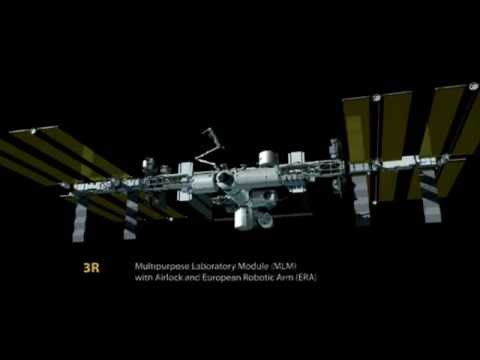The image depicts a sleek, sophisticated mechanical machine set against a dark black background speckled with white dots resembling stars. The primary subject appears to be a multipurpose laboratory module (MLM) with an airlock and European robotic arm (ERA), labeled "3R" underneath. The module is constructed from silver or gray metal and runs horizontally, with straight lines resembling wings or arms extending from both sides. Each arm features four gold or yellow rectangular slats. Central to the machine is a small, circular black component that looks like a camera, and the structure is adorned with various knobs, nuts, bolts, and other mechanical appendages. At the base of the module, there are additional silver rectangular strips and a tubular object with a dark opening at the tip, giving it an intricate and high-tech appearance, akin to a cross between a satellite and a spaceship.